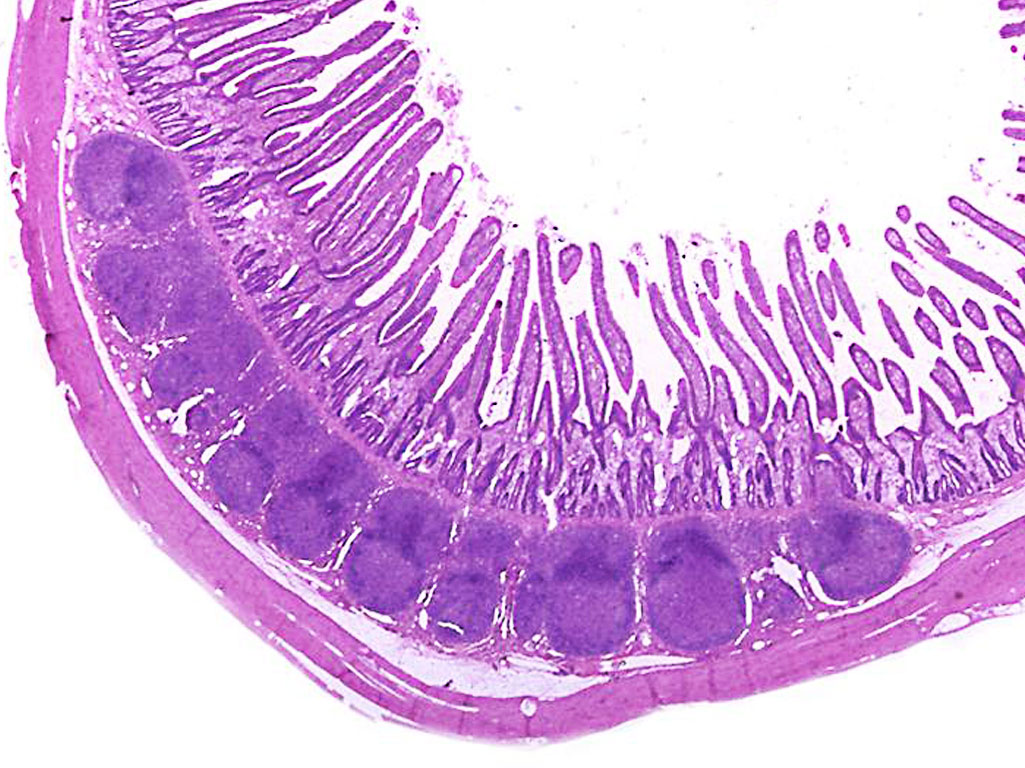This image presents as a detailed and vibrant scientific slide photograph showing a cross-section view of the ilium, part of the gastrointestinal tract. Primarily in varying shades of purple against a white background, the image is meticulously detailed. Floating within the white space, the illustration occupies a square frame without borders, appearing to emerge organically from the blank canvas.

At the top of the composition, the white background dominates, creating a minimalist setting that contrasts sharply with the intricate details below. From this white expanse, lines or streaks of lighter purple descend in a manner reminiscent of raindrops, contributing to a dynamic transition into the more complex structures beneath.

The central focus of the image is a circular formation, with the bottom half of this figure showcasing a collection of dark purple, rounded, rectangular shapes. These are segmented from one another by thinner, lighter purple borders and occasional white gaps, hinting at the layered and cellular nature of the depicted tissue.

Framing this detailed central composition is a thick, irregular, squiggly purple line, adding a slightly whimsical touch that contrasts with the precision expected in scientific documentation. This circular outline encases the heavier purple base within, which supports the entire depiction, lending it an almost organic, child-like simplicity amidst the scientific context. The representation underscores the complexity and beauty of biology, making the microscopic both accessible and intriguingly artistic.